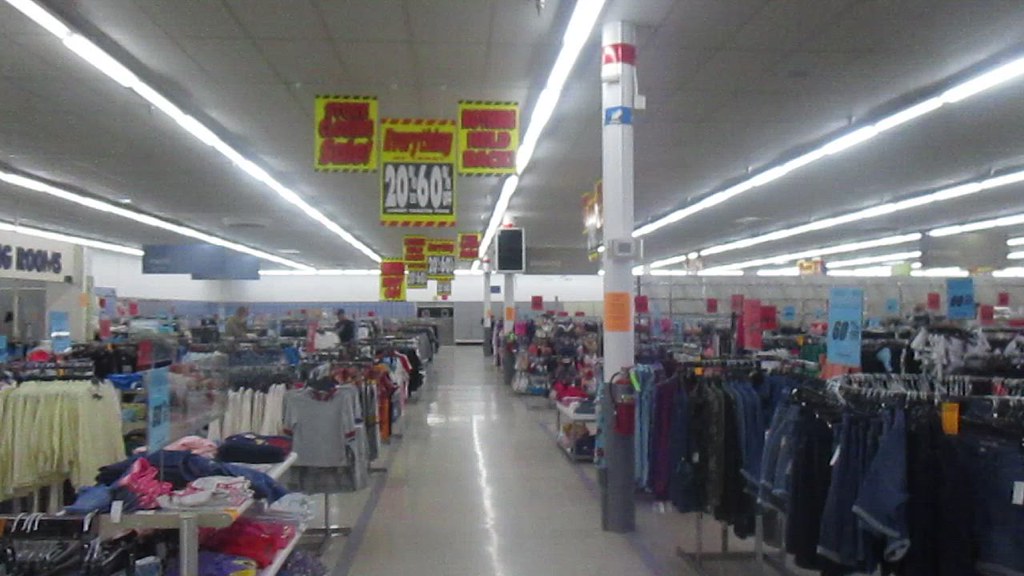This is an interior photo of a retail clothing store taken from within an aisle. The ceiling is lined with fluorescent lights set into ceiling tiles, brightly illuminating the space. Yellow signs with red and white lettering hang from the ceiling, prominently declaring "Everything 20 to 60% off," with similar signs visible further back. The store is bustling with various clothing displays: racks filled with t-shirts, jeans, and jackets, some on straight poles and others on circular racks. The floor is hard white with red lines marking the pathway distinct from the shopping areas. To the left, there's a sign partially visible, likely indicating fitting rooms. Clothing items are arranged in a spectrum of colors: predominantly dark blues are on the right, while a mix of colors is on the left. A standout feature includes an orange sign mounted on a pole. In the very back, an appliance can be faintly seen, hinting at a diverse product range within the store.